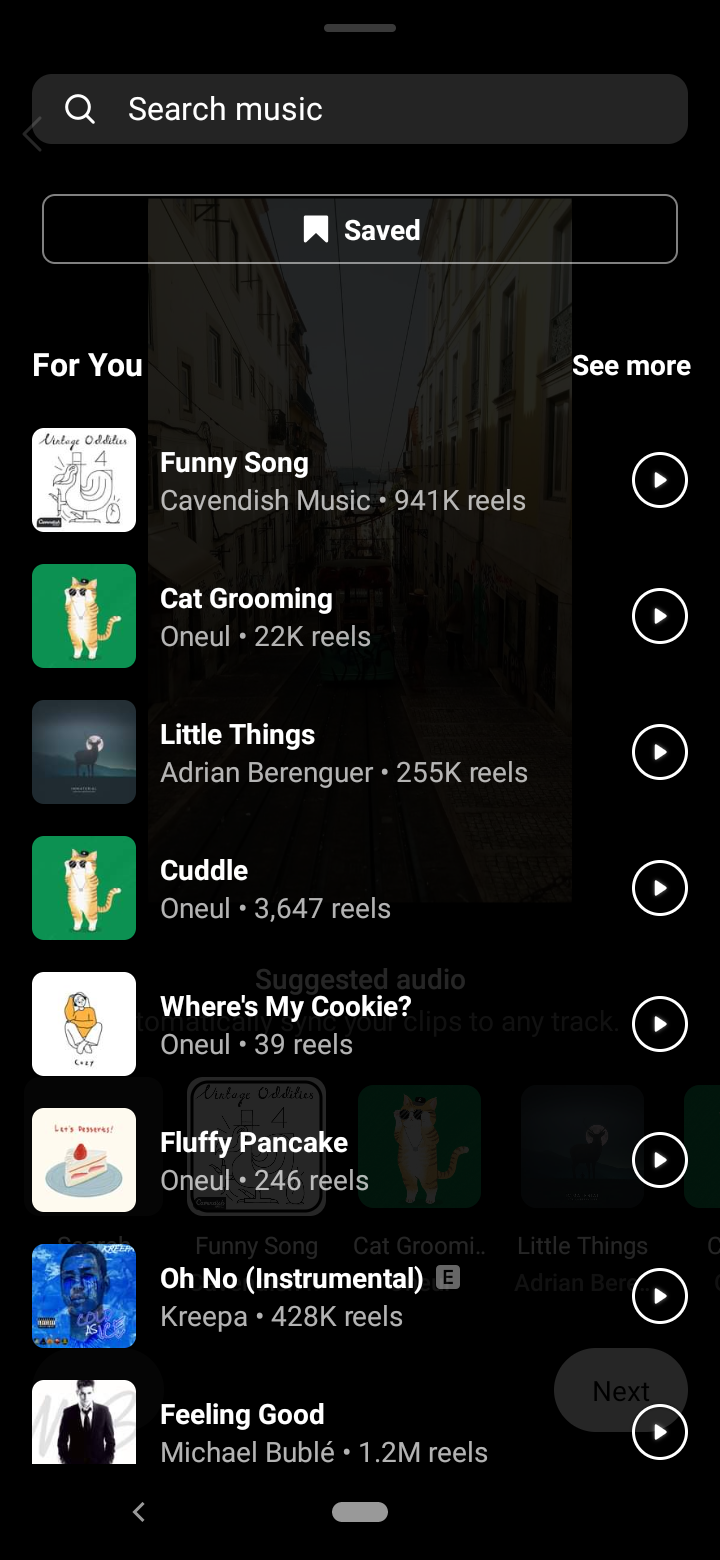The image is a screenshot of the search area within a music website or app interface. At the top, there is a gray search bar with the placeholder text "Search music" displayed inside. Below this, there is a clear bar labeled "Saved," featuring a bookmark icon next to it. On the left side of the screen, the text "For You" is prominently displayed, while on the right side, there is an option labeled "See More." 

The list of songs includes unique and playful titles as follows:
1. Funny Song
2. Cat Grooming
3. Little Things
4. Cuddle
5. Where's My Cookie
6. Fluffy Pancake
7. Oh No (Instrumental) – indicated by a small gray box with an "E" inside
8. Feeling Good